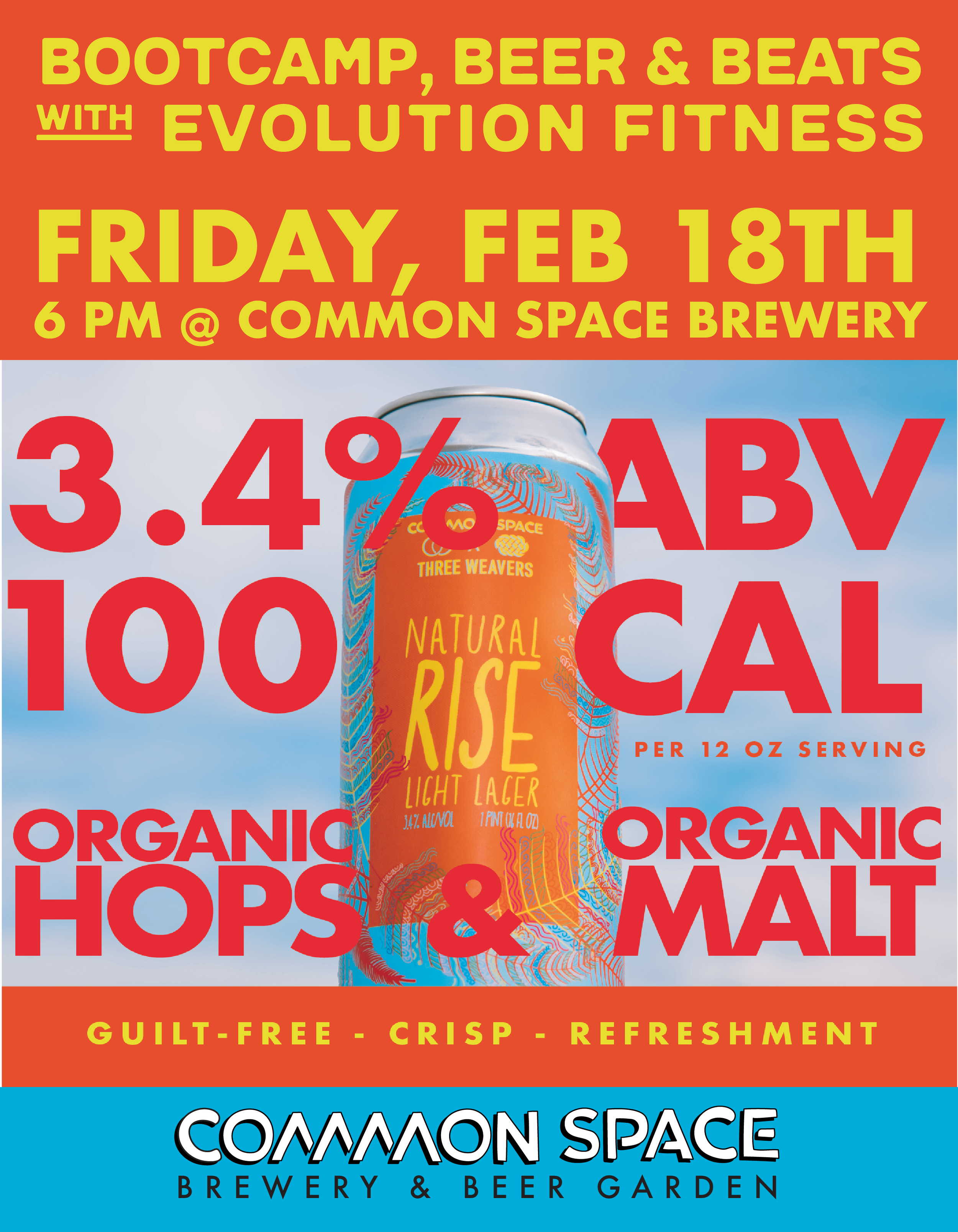This advertisement for Common Space Brewery's "Bootcamp, Beer, and Beets with Evolution Fitness" event on Friday, February 18th at 6 p.m. prominently features a can of Natural Rise Light Lager. The vibrant poster employs a color scheme of red, blue, orange, yellow, black, and white to draw attention. The upper quarter of the image is bold red, displaying the event details. Below, a sky-like background hosts a striking can of beer, adorned with the text "3.4% ABV, 100 CAL per 12 oz serving, Organic hops and organic malt," in large red letters. A red bar beneath the can adds "Guilt-free crisp refreshment," followed by a robin's egg blue bar at the bottom with "Common Space Brewery and Beer Garden" in black text, bordered by white. Intricate details on the can enhance its visual appeal, incorporating a complex background design that mirrors the ad’s dynamic aesthetic.